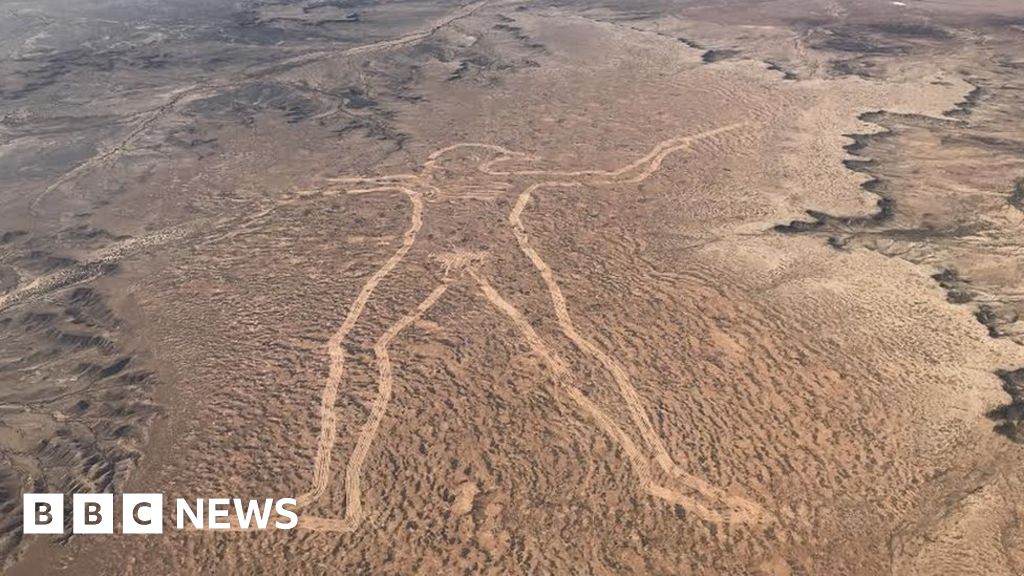The image, likely a photograph from a BBC News report as indicated by the white text in the bottom left corner, appears to be taken from an aerial perspective, possibly from a drone or helicopter. It showcases a vast, barren desert landscape with a striking large-scale design etched into the land. The design resembles a human figure with an eagle's head, stretched out as if making a snow angel in the sand. This human-eagle hybrid figure appears to be holding a staff or wand and is simply an outline carved into the desert terrain. The region near the pelvic area is obscured by a deliberately placed bush, adding an element of modesty. The surrounding area is entirely composed of brown sand, emphasizing the arid, lifeless environment.